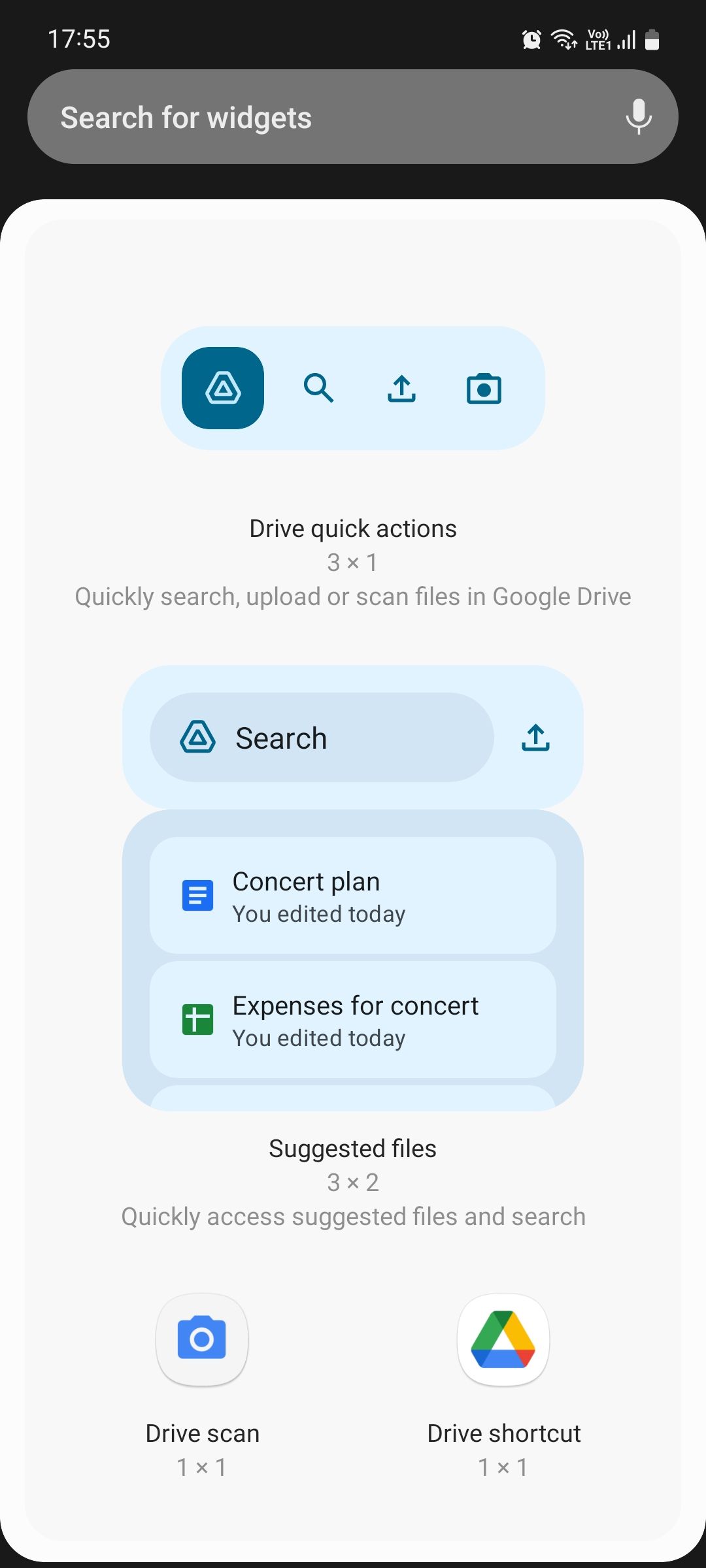In this vertically-oriented rectangular image, we observe a screenshot featuring a predominantly white background with light blue accents. The image begins with a black header at the top. On the left side of the header, the time is displayed as 17:55. Within this black section, there is a search bar labeled "Search for widgets." 

Below the black header and search bar, the background transitions to white, where various light blue rectangular options are present. 

Starting from the top:
1. The first light blue section is labeled "Drive Quick Actions (3x1)." This section allows users to quickly search, upload, or scan files in Google Drive.
2. Beneath that, a search bar is present.
3. Below the search bar, two items are listed: "Concert Plan (edited today)" and "Expenses for Concert (edited today)." 

Next, there is a section labeled "Suggested Files (3x2)," which provides quick access to suggested files and the search function.

Towards the bottom left, we have a "Drive Scan" option (1x1) represented by an image of a camera, suggesting the ability to scan documents directly to Google Drive.

On the lower right, there is a "Drive Shortcut" (1x1), offering a quick link to access Google Drive features.

Overall, the image showcases various Google Drive functionalities, emphasizing ease of access and quick actions.